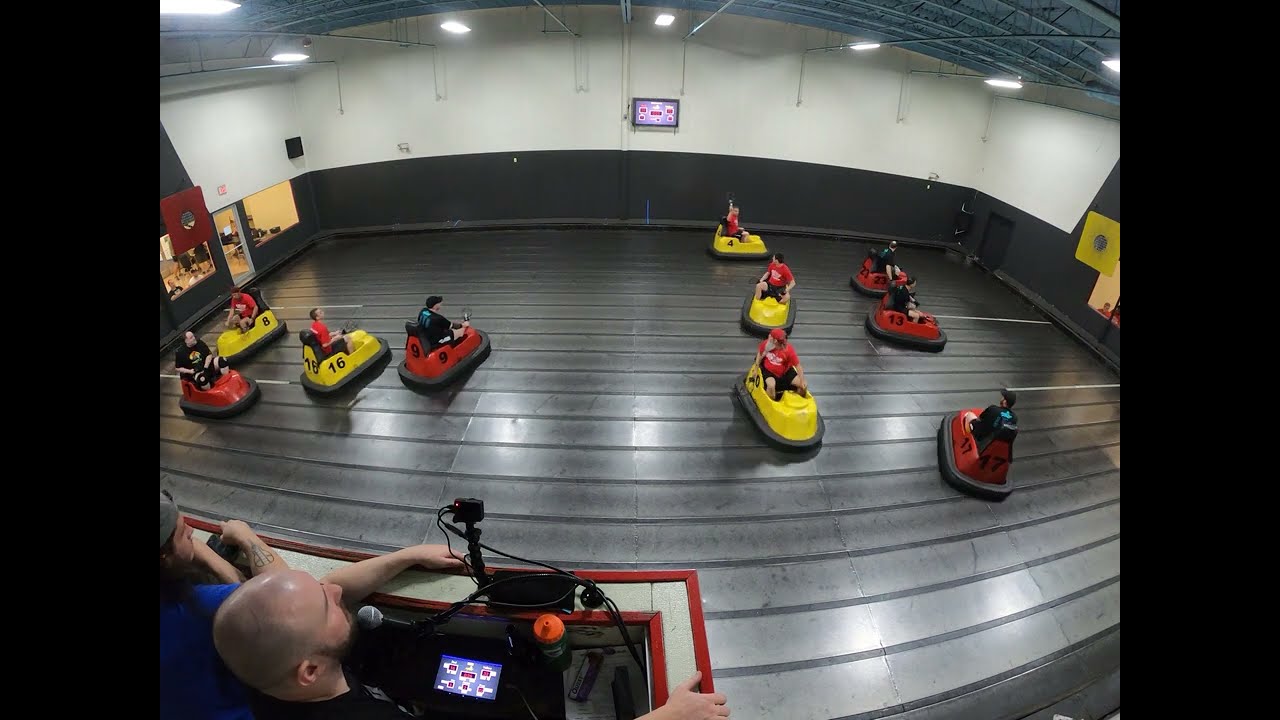The photograph captures an aerial view of an indoor bumper car arena. The arena features a black, rubberized floor and an off-white ceiling with bright white fluorescent lights, illuminating the scene vividly. The room's walls are white above a black section, and there's a possible scoreboard visible in the background. The track is occupied by approximately 10 bumper cars—five red and five yellow—each with distinct numbers like 80, 16, 9, and 13, scattered across the floor. The drivers of the yellow cars are dressed in red shirts, while those in the red cars wear black shirts.

In the foreground, there's a booth housing two men. One man, who is bald and bearded, sits in front of a microphone, likely the commentator, and is flanked by a digital display or a computer. He is wearing a dark shirt. Beside him, another man in a blue t-shirt and a hat observes the scene. The bumper cars appear stationary, possibly awaiting instructions from the commentator. The overall image is clear, high-quality, and brightly lit, showing the details of the arena and its occupants vividly.